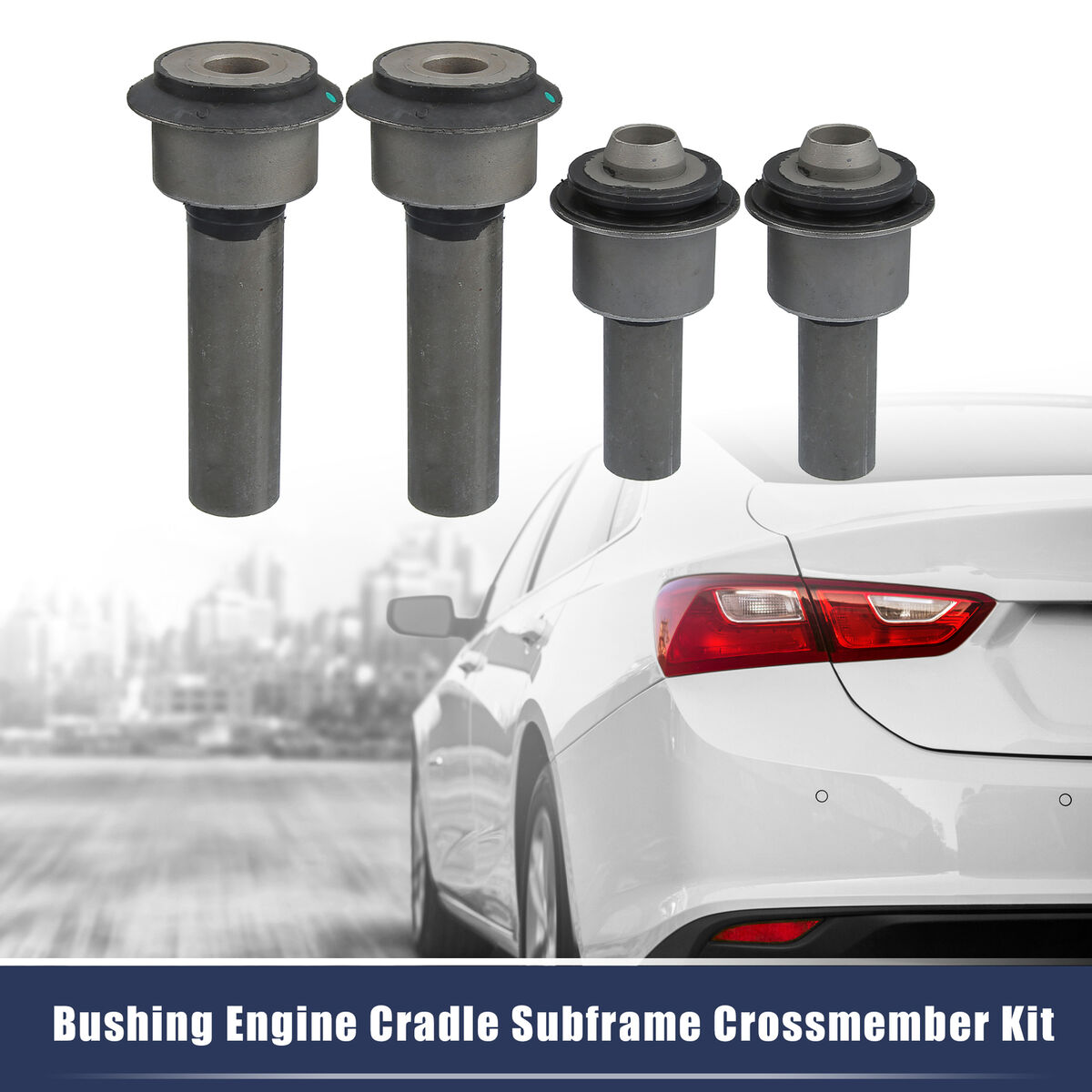The image is an advertisement for car parts, specifically a "bushing engine cradle subframe crossmember kit." Dominating the foreground is a detailed close-up of a white sedan, its left side and distinct red taillights clearly visible as it drives down a long stretch of road. The background features a black-and-white cityscape silhouette, giving a stark contrast to the colorful car. Above the car, four dark gray automotive bolts—two long ones on the left and two shorter ones on the right—are prominently displayed. These bolts, part of the kit being advertised, are designed with circular rods and holes for easy installation. The advertisement's title is prominently displayed at the bottom of the image in bold white letters against a dark blue banner. The overall scene blends elements of color and monochrome to draw attention to the car and the featured parts.